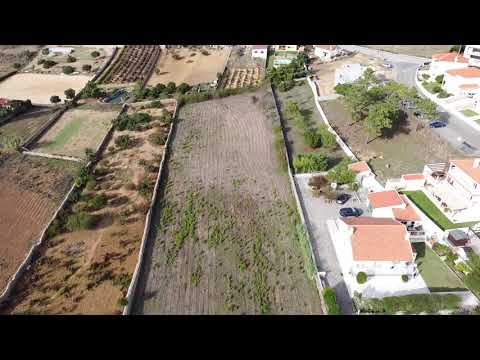A high-angle drone shot captures a picturesque aerial view of farmland divided into various large rectangular and square plots, each characterized by distinct vegetation patterns and color variations. Some plots appear nearly bare, indicating an early or late season, while others exhibit rows of green growth, possibly grapevines, alongside patches of brown soil and sparse greenery. The fields are irregularly shaped yet predominantly rectangular, with some wider fields segmented into smaller rectangles. In the center, a large rectangular field is bordered by fencing, with patches of light green and brown hues. On the left, narrow strips of orange-green land contrast with strips featuring more significant vegetation, potentially low trees. White-walled buildings with red sloped roofs scatter along the right side, some nestled on a hillside alongside a roadway network where cars are visible, reinforcing the image of a cultivated, yet residential, agricultural landscape.